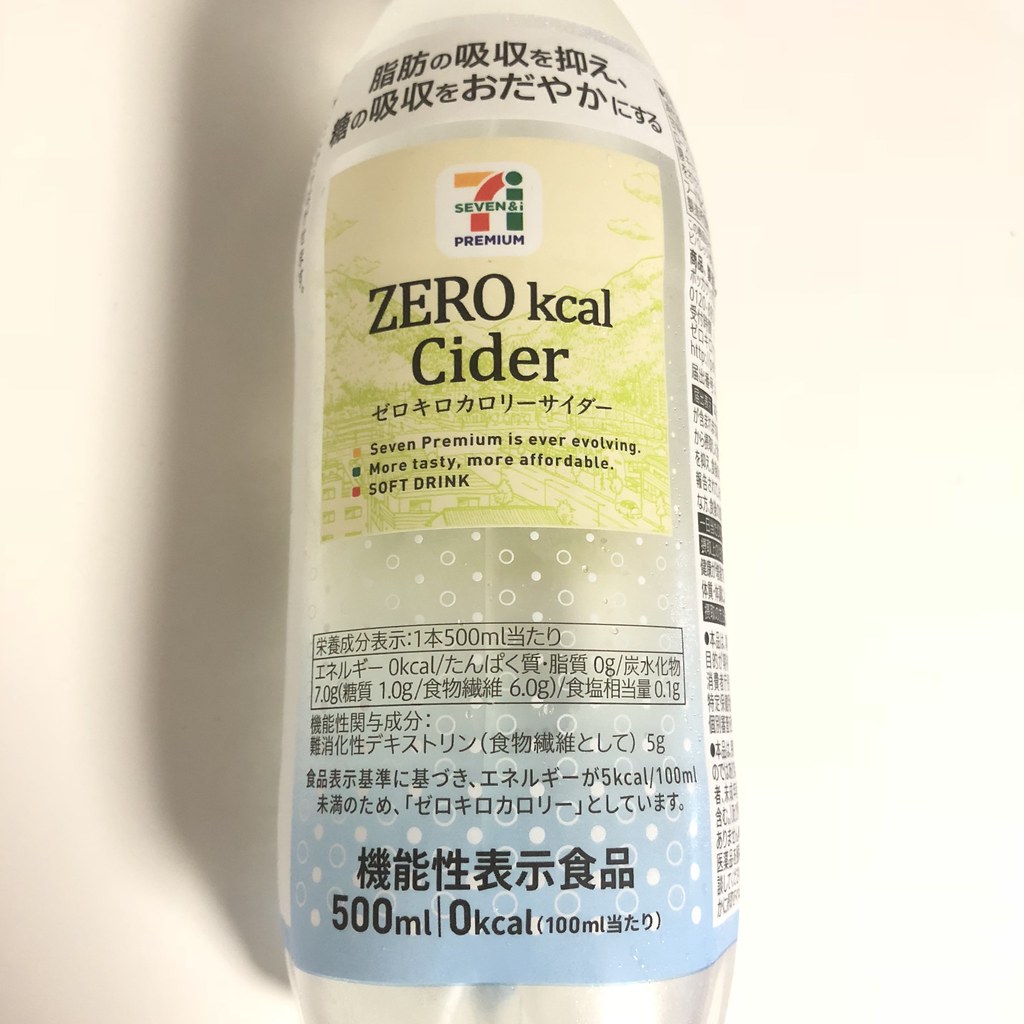The image displays a clear plastic bottle of cider set against a white background, casting a shadow to its left. The bottle prominently features Japanese text, suggesting it is a product from Japan, potentially linked to the 7-Eleven brand. At the top of the label, a green section displays the "7 and I Premium" logo, reminiscent of the 7-Eleven emblem. Below that, the label notes the drink as “Zero Kcal Cider,” indicating it has zero calories. Additional details include a white label with black Japanese characters at the top and a blue portion at the bottom, adorned with white bubbles and more Japanese text. The bottle holds 500 milliliters of clear liquid and the label emphasizes the product’s evolving nature with the phrases “7 Premium is ever-evolving, more tasty, more affordable.” A glimpse of the nutritional information can be seen on the side, providing further details in Japanese.